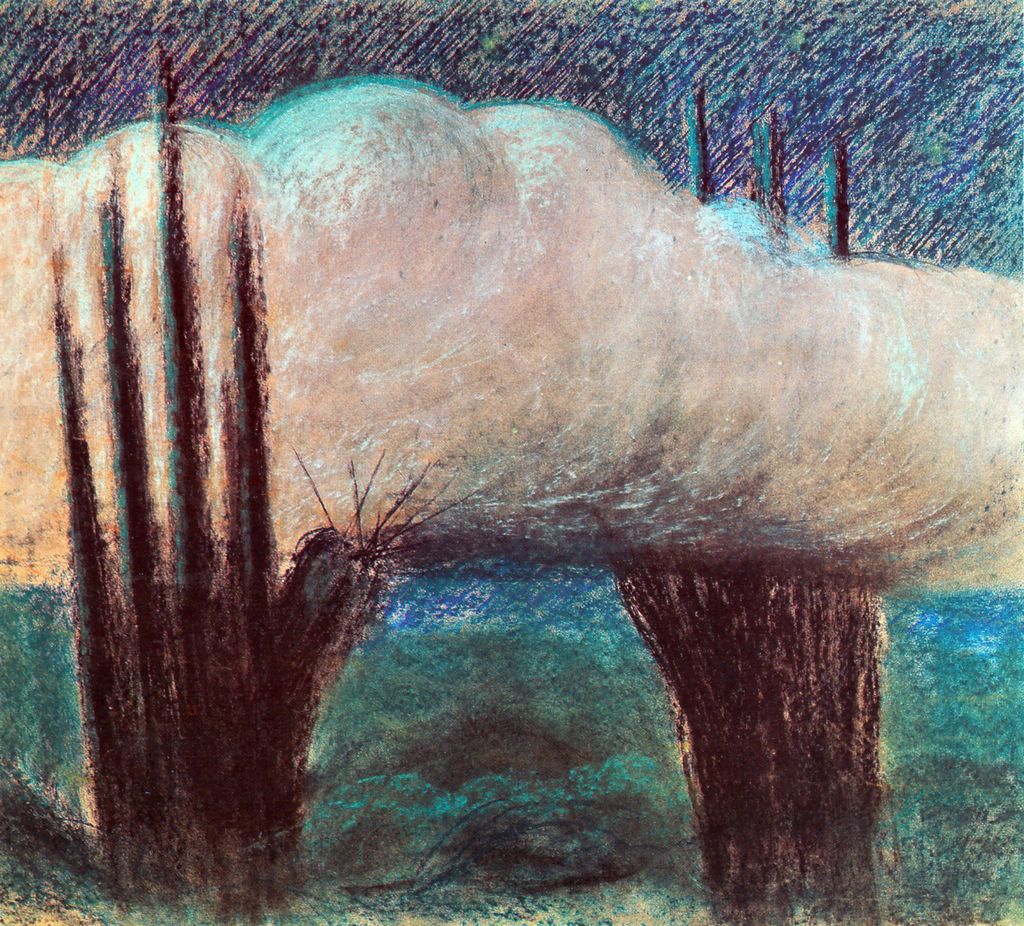The image depicts an abstract natural scene, possibly created with pastels or a similar medium. Dominating the scene are two dark, tree-like structures or cacti with large, spiky branches that stretch upwards, somewhat resembling elongated, stylized hands. The larger trunks and offshoots of these structures are rendered in black and brown. Above and behind these structures, a massive, whitish-gray cloud spans the scene, obscuring parts of the sky and crossing through the branches. The sky itself transitions from a dark blue at the top to a lighter blue and green nearer the horizon. The ground below features a blue-green hue. The overall impression is of a surreal, almost mystical landscape, blending stark, skeletal plants with a dramatic, sweeping sky.